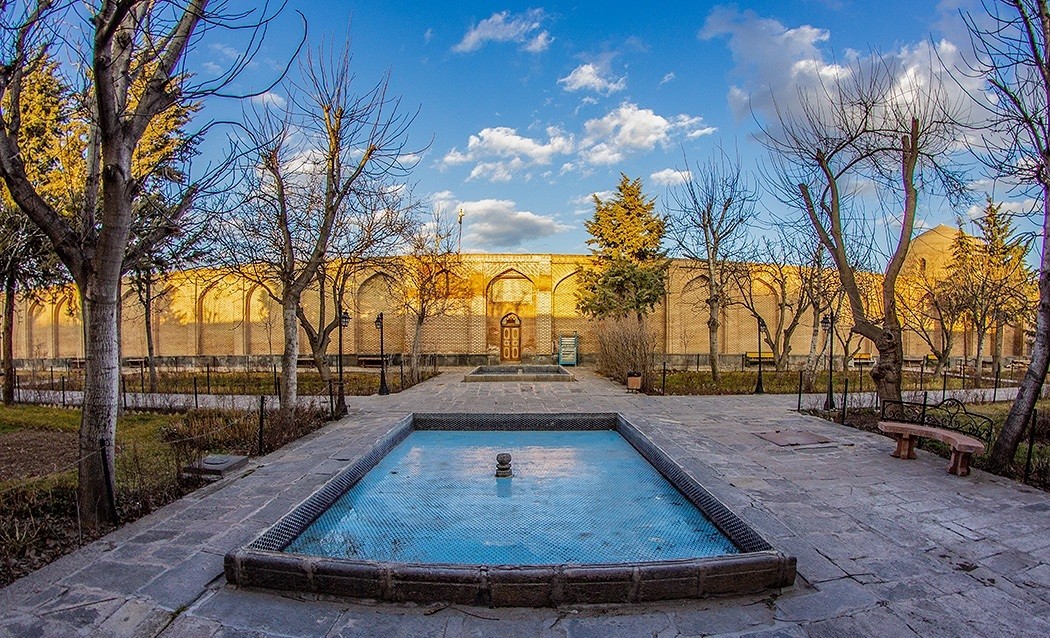The image captures a serene public courtyard, likely photographed during dawn or dusk, indicated by the shadows and the soft sunlight. At the center of the scene is a bright blue, rectangular pool, about a foot deep, bordered by a low stone wall. In its middle, there's a cylindrical object resembling the base of a fountain, currently inactive. Surrounding this central pool is a flat patio surface, leading up to another square pool of water ahead.

To the right, a curved, stone and concrete bench adds a place for respite. The image suggests it's fall, as many of the trees, both in the foreground and background, are bare or have sparse leaves. The sun appears to be setting or rising from the top left, casting a golden hue on a large wall in the background. This wall, stretching across the width of the image, is comprised of light brown or golden-yellow bricks with decorative arches, and partly illuminates while the rest remains in shadow.

Flanking the courtyard are patches of green grass interspersed with dirt, and further back, partially obscured by trees, there's a glimpse of a tower. The sky above is partly cloudy, contrasting with its vivid blue hue, encapsulating the tranquil and historical essence of this public space.